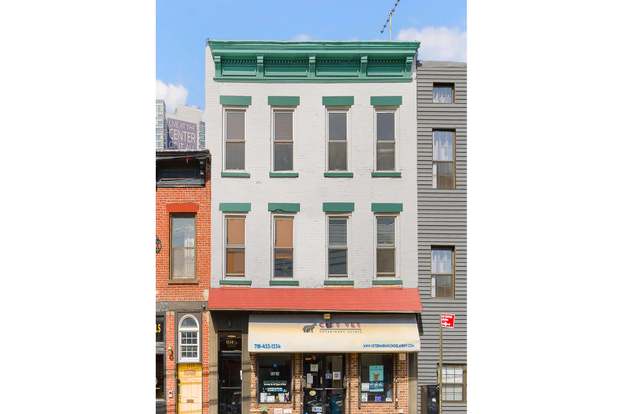The image depicts a light gray, three-story building nestled between a shorter, reddish brick building on the left and a dark gray, metal-panel building on the right. The central building features emerald green accents framing each window and is topped with intricate green ornamental details in a Greek architectural style. Above the building rises a TV antenna against a backdrop of a blue sky with fluffy white clouds. The ground floor, constructed of brown brick, houses a storefront distinguished by a red and a yellow canopy. This storefront includes a single doorway flanked by two large glass windows. The adjacent buildings partially frame the central structure, adding a sense of enclosure and highlighting the distinctive color contrast between the reddish brick on the left and the horizontal gray siding on the right.